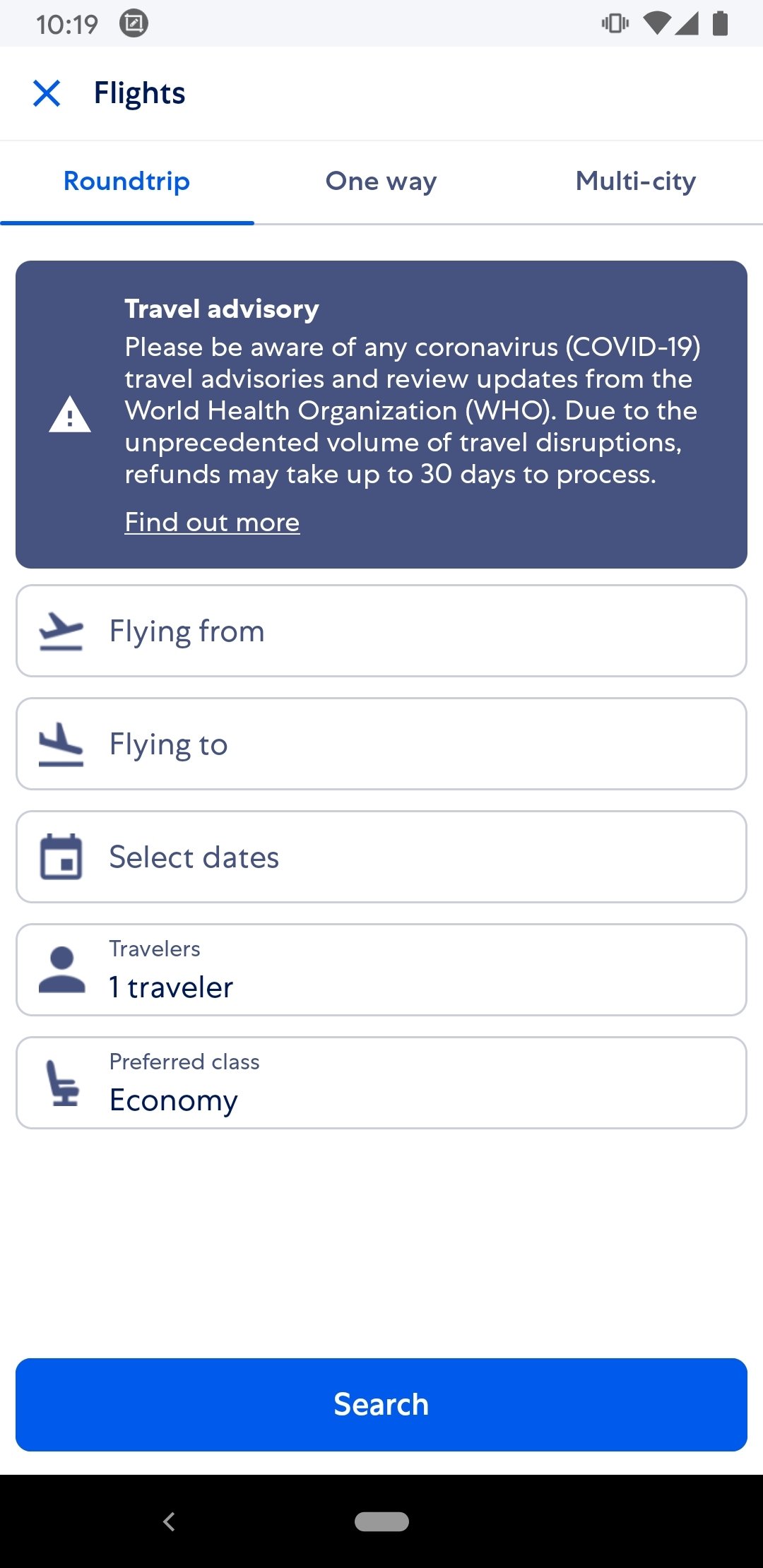This is a detailed and cleaned-up descriptive caption for the provided image:

---

The image displays a mobile phone or tablet in a vertical orientation, showcasing a travel booking app interface. At the top of the screen, within a gray border, the current time is shown as 10:19. On the left, there is a circular icon featuring a box with a pencil inside. On the right-hand side, there are icons for vibration mode, full data signal, Wi-Fi connection, and battery status.

Beneath this, the app interface presents a white background with a blue "X" icon on the left, followed by the word "Flights" in navy blue font. Next, there's a section allowing users to choose their trip type: "Round Trip," "One Way," or "Multi-City," with "Round Trip" currently selected. Directly below, a prominent blue box displays a "Travel Advisory," alerting users to be aware of coronavirus (COVID-19) travel advisories and to review updates from the World Health Organization. It advises that due to an unprecedented volume of travel disruptions, refunds may take up to 30 days to process, and provides a link to "Find out more."

Below the advisory, the interface lists input sections labeled: "Flying From," "Flying To," "Select Dates," "Travelers" (currently set to one traveler), and "Preferred Class" (currently set to Economy). At the bottom of the screen, there is a blue rectangular button labeled "Search" in white text. The bottom-most part of the image features a black bar with a gray back arrow on the left side and an icon for the homepage on the right.